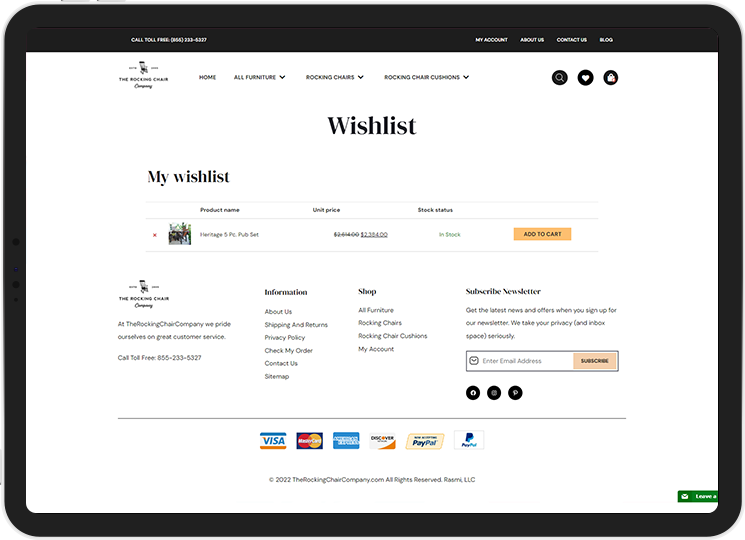This image depicts a stylized screenshot of a website, showcased within a digital drawing of a tablet. The tablet, featuring a black outer frame, has three discernible buttons located on the top and side edges. The screenshot, although integrated within the tablet frame as if it were a real screen, lacks realistic detail and exhibits low image quality, making smaller elements difficult to read.

At the top of the screenshot, there is a black rectangular header containing a navigational menu with white text, listing options such as "My Account," "About Us," "Contact Us," and "Blog." Below this primary menu, the main web content is presented on a white background, featuring a secondary navigational menu. This secondary menu, in black text, includes categories like "Home," "All Furniture," "Rocking Chairs," and "Rocking Chair Cushions."

The central focus of the image is a wishlist section of the website, where users can save items they are interested in purchasing. Towards the bottom, a site navigation map is visible, accompanied by a footer displaying various brand icons representing accepted payment methods.